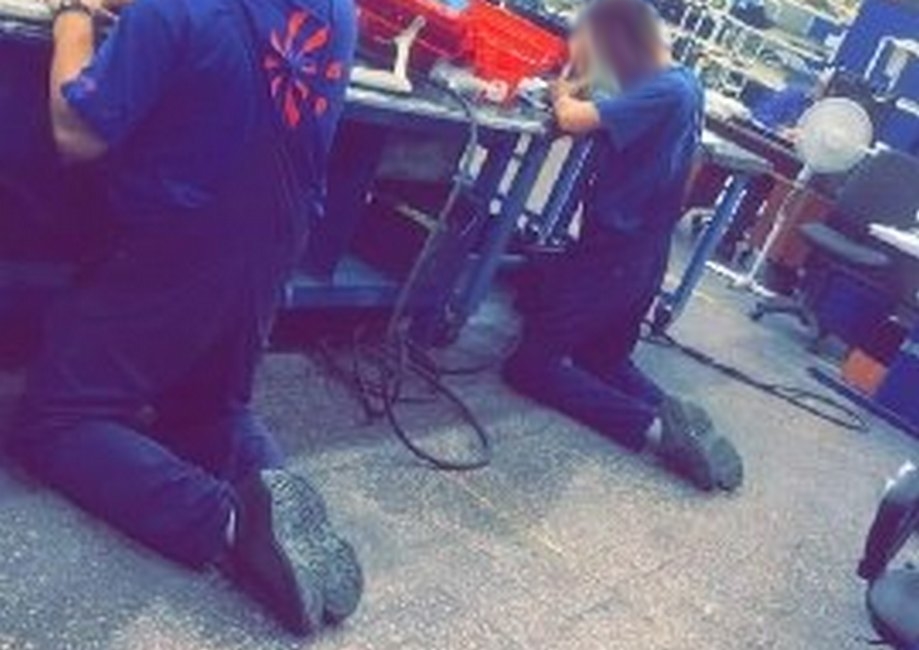The image depicts two men in blue overalls and light blue t-shirts, kneeling on the floor as they work diligently at a long metal workbench in front of them. The workbench appears to be composed of several sections joined together, creating an extensive workspace. On the workbench, there are several red plastic boxes, which seem to be toolboxes containing various pieces of equipment. Various cables run from the floor up to the workbench, indicating a likely usage of electronic or electrical tools.

In the background, beyond the two men, a fan mounted on a tripod can be seen, noticeably turned on to provide ventilation in the room. Nearby, there is also a swivel chair positioned close to the fan. Intriguingly, one of the men's faces is blurred in the image, making it impossible to identify him. Both men have bare arms visible, suggesting a potential for manual and perhaps strenuous physical labor.

Despite their active engagement, the men's kneeling position on the hard floor appears notably uncomfortable, hinting at the physical strain such a posture might entail if maintained for extended periods. This detail highlights the challenging working conditions captured in the image.